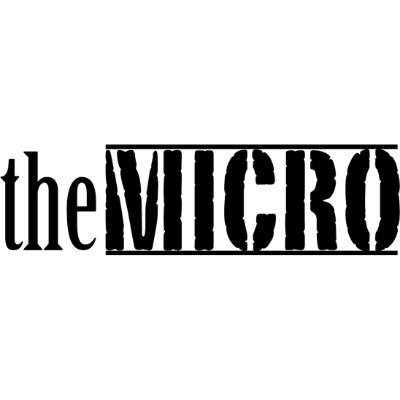The image features a simple yet striking design of black text on a completely white background, creating the illusion of the words floating in a white void. The text consists of two words: "the" and "MICRO." The word "the" is in lowercase, using a tall, thin, and elegant black font that appears professional and refined. Positioned to the left, it contrasts sharply with the word "MICRO," which is in all capital letters, utilizing a thick, dark, stencil-style font. This bold font has random white lines cutting through the letters, with solid black lines both above and below, giving it the appearance of having been spray painted through a stencil. Together, these divergent styles—minimalistic yet impactful—suggest a tagline or brand name, potentially for an advertisement or a clothing line.